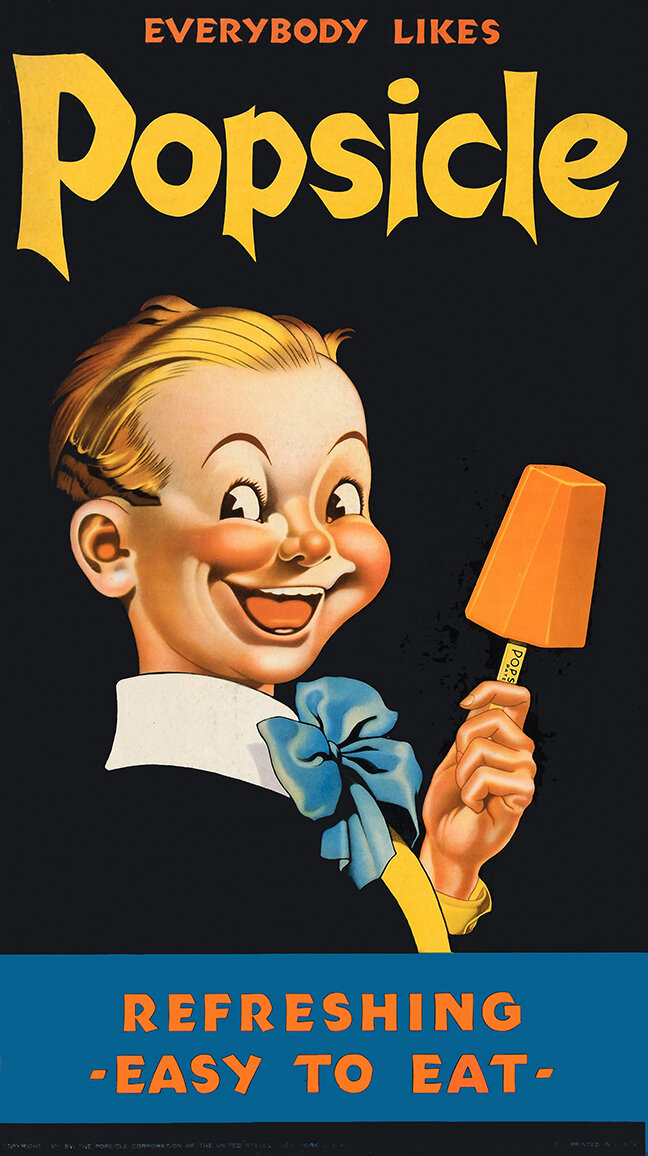The poster depicts a cheerful young boy with slicked-back, orangey-blonde hair and red cheeks, prominently smiling and holding an orange cream popsicle upright in his left hand. The boy is drawn wearing a blue bow tie over a white shirt and suit coat. The background of the poster is predominantly black, transitioning into a blue bar at the bottom. At the top of the image, bold orange text reads "Everybody Likes," followed by the word "Popsicles" in large yellow letters. The blue bar at the bottom features the text "Refreshing, Easy to Eat" in orange. This vintage-style artwork has a nostalgic charm, emphasizing the delight of enjoying a simple, refreshing treat.